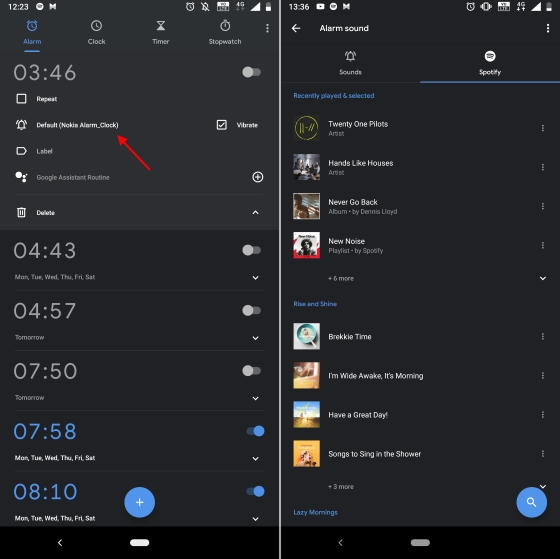The image consists of two adjacent smartphone screen captures. The first screen capture displays an alarm clock schedule, indicating a current time of 3:46, alongside a series of previously set alarms. These alarms include times of 4:43, 4:57, 7:50, 7:58, and 8:10. Notably, the 7:58 and 8:10 alarms are activated, appearing in a different color or with an 'on' indicator.

The second screen capture features a music playlist, containing thumbnails that resemble album or CD covers. Each thumbnail is accompanied by the song title and artist name, though the text appears significantly small and challenging to read. The playlist seemingly includes multiple entries, suggesting a variety of songs or MP3s compiled by the user.

Both screens are displayed in night mode, characterized by a black background, which facilitates readability in low-light environments. The choice to juxtapose these particular screens—one representing the user's daily alarm schedule and the other their musical preferences—may provide a glimpse into their morning routine or personal habits.